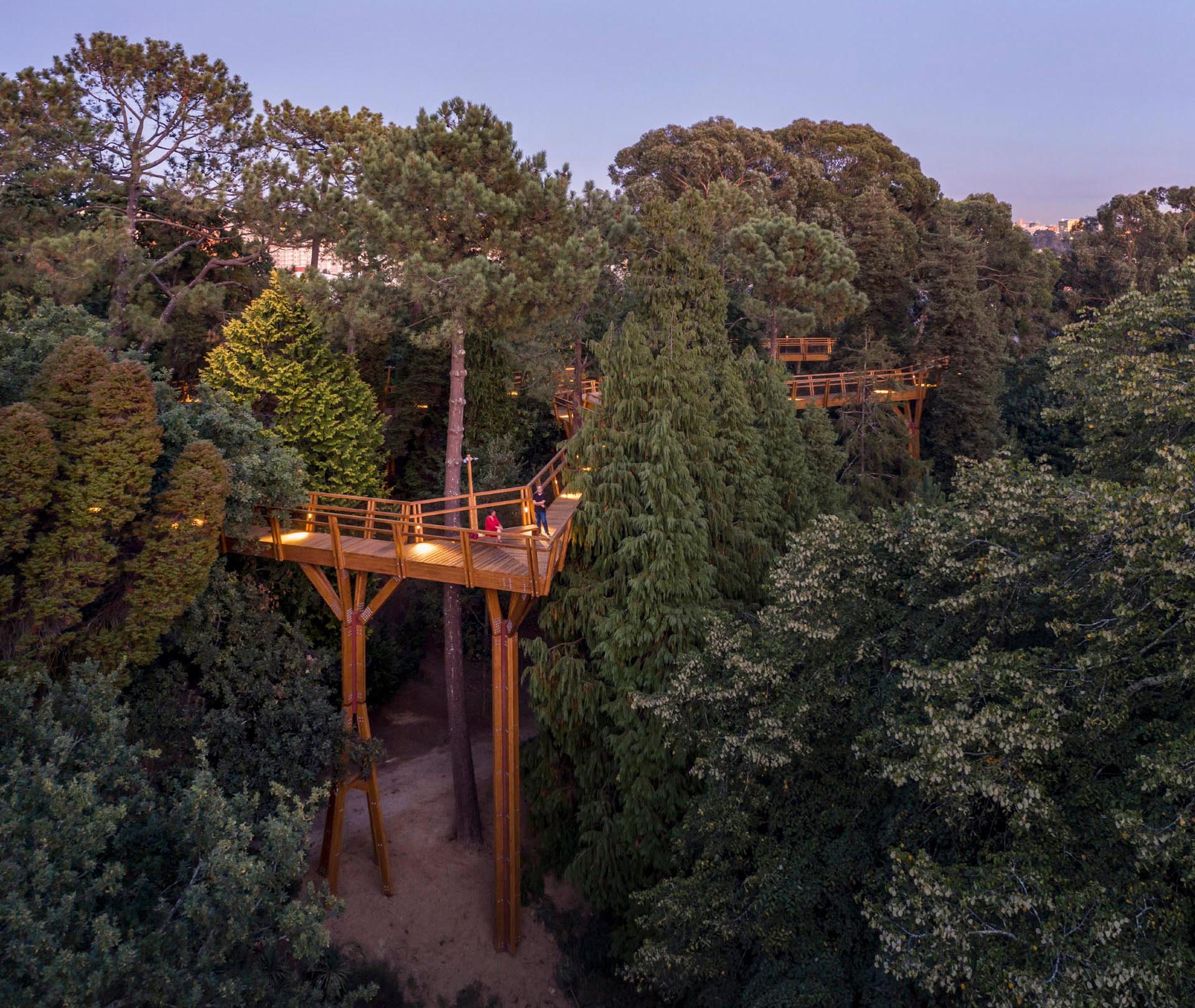The photograph captures a stunning scene of a heavily forested area characterized by very tall trees, both pine and deciduous, with a uniquely constructed wooden walkway on stilts weaving its way through the treetops. This elevated path, standing approximately 20 to 40 feet high, is made from medium brown, possibly stained wood, and extends far into the distance, zigzagging between and sometimes under the treetops. The sky, tinged with purplish hues suggesting dusk, adds to the serene ambiance. Some trees have been trimmed to make space for the walkway, while small clearings accommodate the strong, supportive stilts. The ground below is scattered with sand and pine needles. In the foreground, a couple of people are seen standing at the corner of the walkway, peering out over the bamboo-like railings. The walkway is adorned with lights to guide visitors, and in the distance, a city skyline is faintly visible, just peeking through the canopy. This unusual and beautiful structure might be part of a resort, offering a breathtaking view and a unique experience of walking among the treetops.